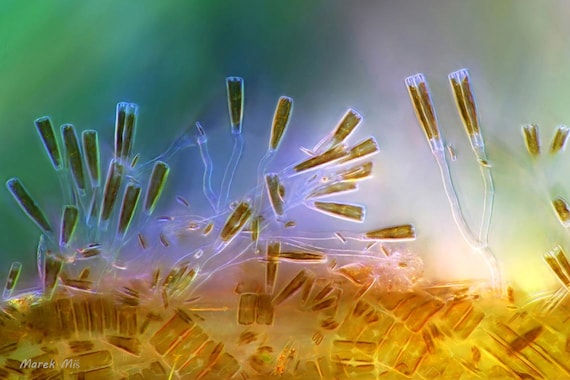The image is a highly magnified photograph, possibly botanical or cellular in nature, resembling something viewed through a microscope. Dominating the foreground is a collection of golden-yellow, rectangular forms with a plastic-like sheen, arranged closely together in an irregular pattern. Emerging from this cluster are translucent, almost clear, extensions that fan out like delicate, tubular structures with golden-yellow, rectangular ends, resembling organic "champagne glasses." The background is a blur of colors, featuring shades of green, purple, and pink, creating a vivid and abstract aesthetic. In the bottom left corner, the name "Merrick Mis" is inscribed in white.